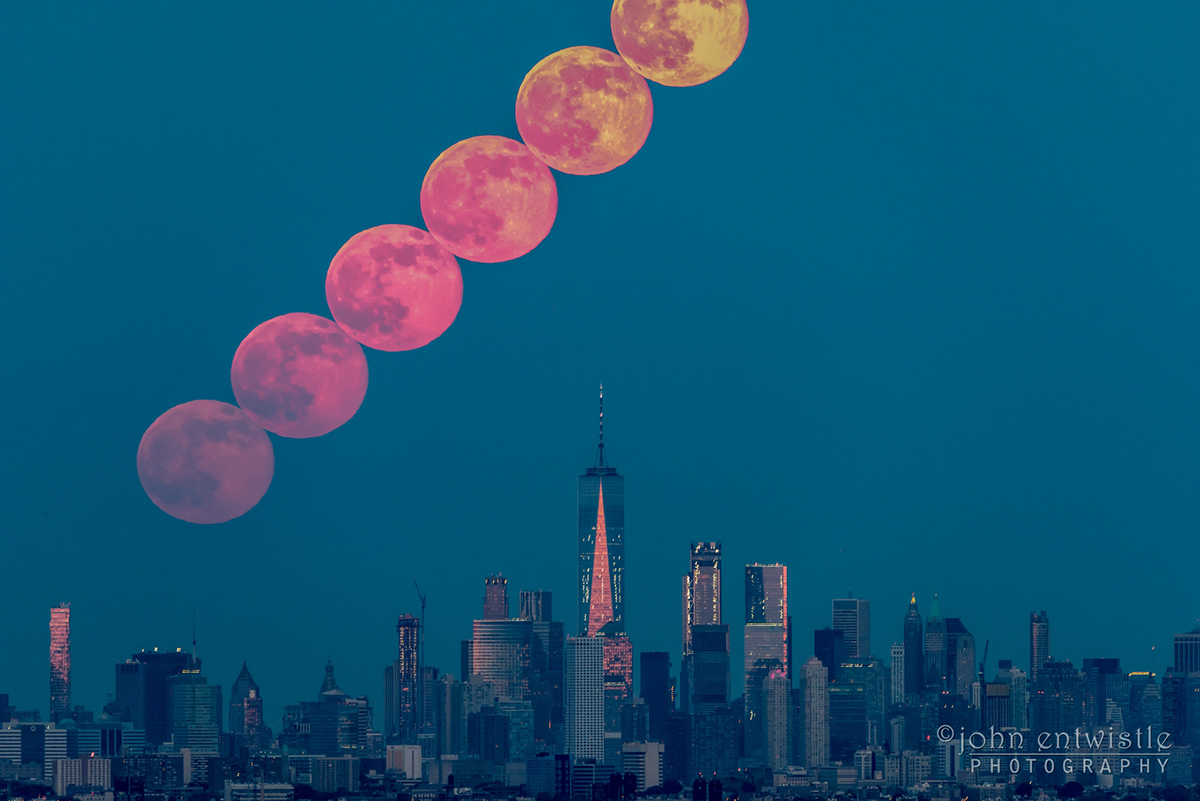A full-color, professionally taken photograph, captured by John Entwistle Photography, showcases a bustling cityscape at night, possibly New York City, recognizable by its iconic skyscrapers. The composition features multiple tall and short buildings, with one prominent skyscraper adorned with a needle-like spire and an illuminated triangular section. The city lights glimmer brightly against the blue night sky, adding to the urban allure. Dominating the upper portion of the image is an artistic representation of the full moon—orange in hue—appearing six times in a sequence from the lower left to the upper right, creating a captivating, almost infrared visual effect. The photograph, presented in a rectangular format with the longer horizontal edge, creatively blends architectural splendor with celestial beauty, marked by the photographer's watermark in the bottom right-hand corner.